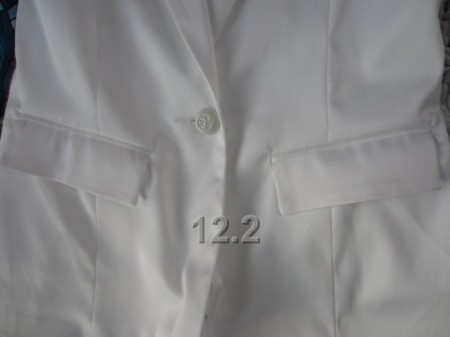In the image, dominating the frame is a pristine white garment, which appears to be a jacket typically worn by a nurse or doctor, or possibly a vest with a satin-like, possibly silky texture. The garment has a single white button in the top center, securing the left and right sides together. Two loose flaps cover pockets on both the left and right sides, with visible stitching outlining each pocket. The background of the image is mostly black, providing heavy shadowing that accentuates the stark whiteness and subtle shine of the fabric. Towards the bottom center of the garment, the white letters "12.2" are prominently displayed in a transparent, blocky font.